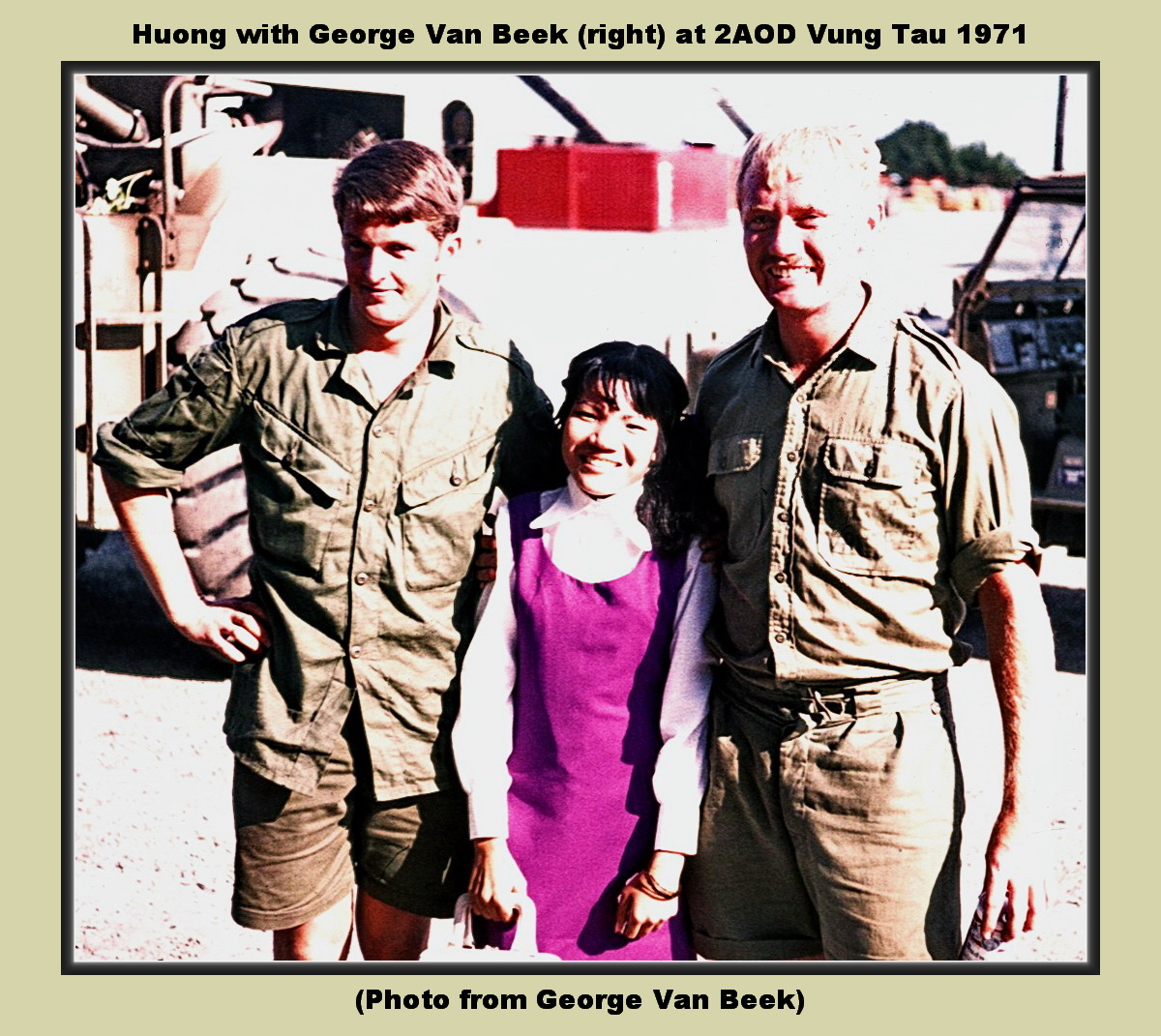This vintage photograph from 1971 shows three individuals posing side-by-side, framed by a light cream-colored border. The man on the right wears a light green button-up shirt with rolled-up sleeves and matching pants. He has blonde hair, a slight glare on the side of his head, and a cheerful expression as he holds a can of beer in his right hand. The young girl in the middle, with dark black hair, beams a smile. She is dressed in a pink shirt under a purple dress and wears bracelets on her right wrist while holding her hands together in front. On the left, another man, this one with light brown hair, sports a light green button-up shirt also rolled to the elbows and matching shorts. He has his left hand on his hip and a shadow cast on the left side of his face with light glaring off the right side. The picture, taken by George Van Beek, has the inscription at the top: "Home with George Van Beek at 2AOW Vung Tau 1971," with "Photo from George Van Beek" written underneath. Army vehicles appear in the background, hinting at the setting.